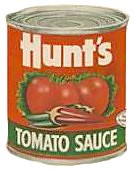The image showcases a vintage or computer-generated depiction of a can of tomato sauce, prominently featuring the Hunt's brand. The can itself is primarily red and displays the brand name "Hunt's" in bold, white letters with an apostrophe S. The top-left edge of the can appears slightly dented, adding an element of wear to the item. 

Front and center on the can's label is an arrangement of two lettuce leaves, each topped with a plump tomato. Beneath this, three chili peppers—two green and one red—are prominently displayed, adding a touch of vibrancy to the design. 

The words "Tomato Sauce" are printed on a green banner across the can, with the letters in white, creating a clear contrast against the background. On the right upper side of this green banner is a small, white oval containing text, but the letters are too small and blurry to make out the writing clearly. The overall aesthetic suggests a blend of vintage design elements with modern visual techniques, emphasizing the product’s freshness and appeal.